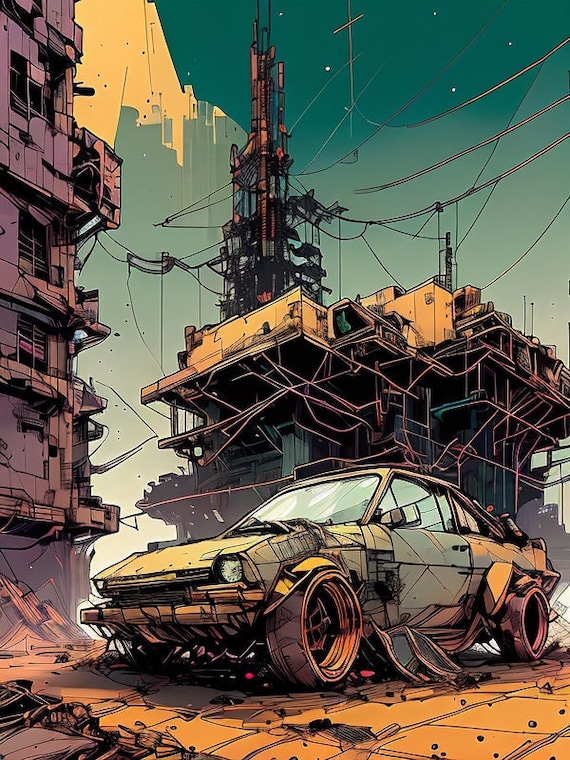This digital artwork portrays a post-apocalyptic, cyberpunk-inspired cityscape with a distinct cartoon or anime style. Dominated by a muted palette of teal blue, orange, and gray, the piece features a central wrecked vehicle that appears both old and futuristic, displaying a greenish, teal hue with visible cracks and a crushed front end. The car, seemingly devoid of wheels, resides on an orange-tiled ground with some tiles dislodged, adding to the scene's overall sense of disarray. In the backdrop, two dilapidated buildings with visible steel beams and attached wires stand against the light teal sky, their structures severely damaged as if by a past bombing. The scene is further accented by dark gray and purplish buildings outlined in the distance, all contributing to the impression of a world marked by significant wear and tear.